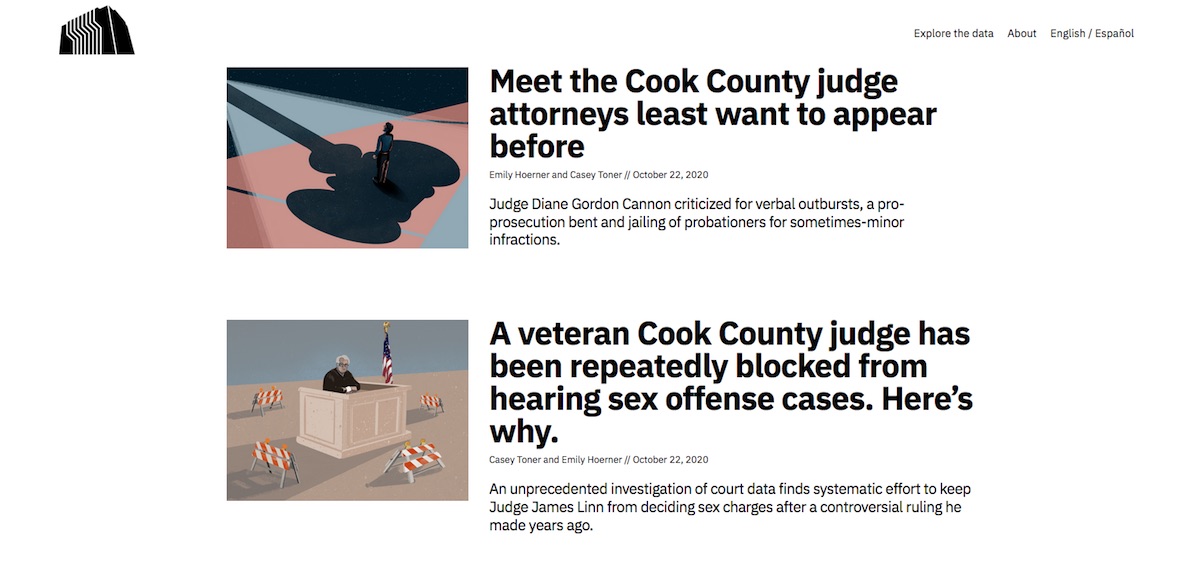Here's a detailed and cleaned-up descriptive caption:

---

Screenshot of a news-related website featuring two highlighted articles. The top left corner displays a black logo, and towards the right, there are options to "Explore Data About" and language choices between English and Español.

1. **Upper Article:**
   - **Image**: A graphic of a gavel casting a shadow.
   - **Title**: "Meet the Cook County Judge Attorneys Least Want to Appear Before"
   - **Authors**: Emily Horner and Casey Toner
   - **Publication Date**: October 22, 2020
   - **Summary**: Judge Diane Gordon Cannon is criticized for her verbal outbursts, a pro-prosecution bias, and her tendency to jail probationers for minor infractions.

2. **Lower Article:**
   - **Image**: A photograph of a judge sitting at a bench.
   - **Title**: "A Veteran Cook County Judge Has Been Repeatedly Blocked from Hearing Sex Offense Cases. Here's Why"
   - **Authors**: Emily Horner and Casey Toner
   - **Publication Date**: October 22, 2020
   - **Summary**: An in-depth investigation of court data reveals a systematic effort to prevent Judge James Lim from adjudicating sex offense cases following a controversial ruling he made years ago.

---

This caption provides a comprehensive overview of the website screenshot and the content of the featured articles.